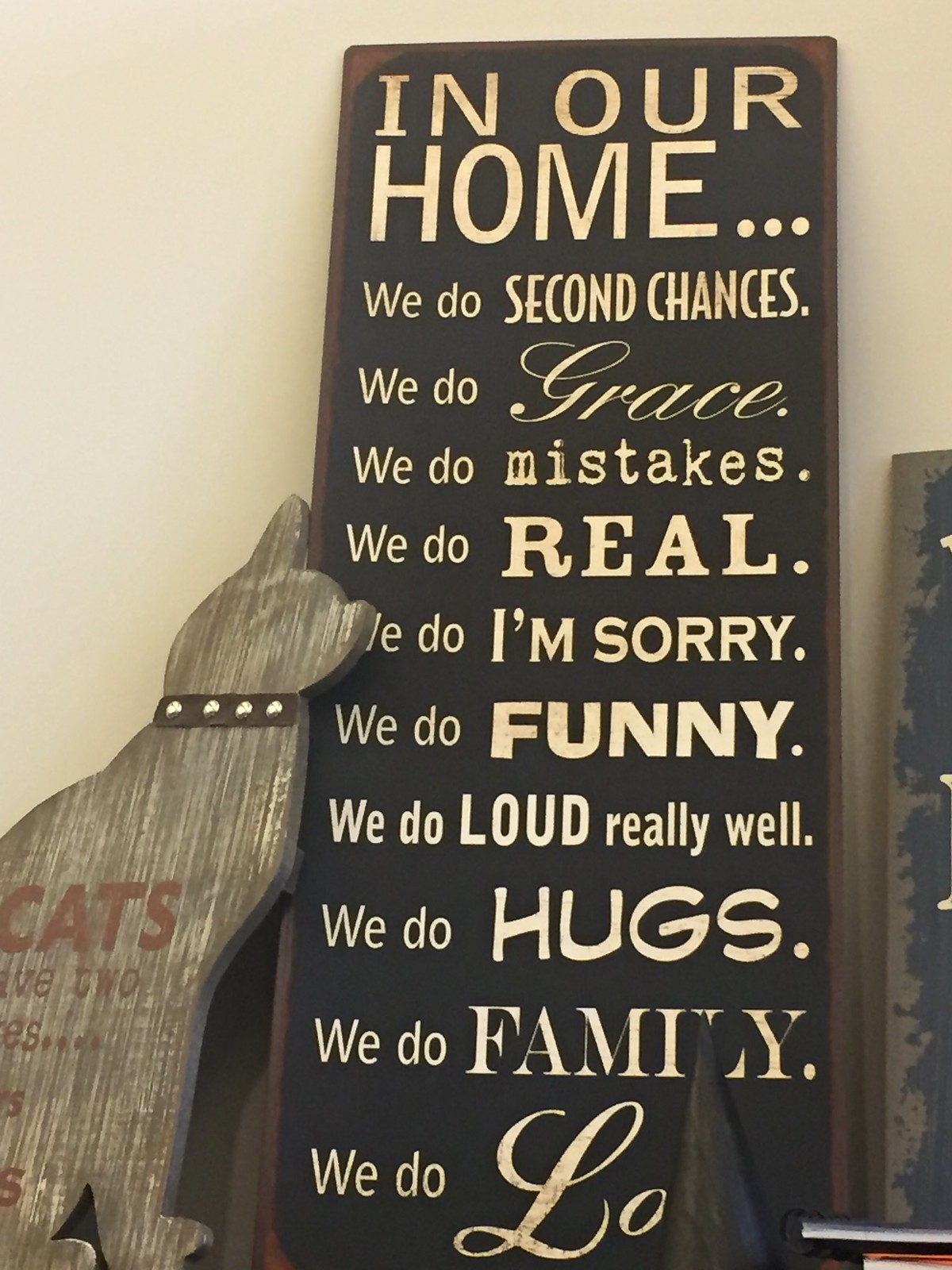The photograph depicts a cozy indoor scene featuring two pieces of wall art displayed against a beige wall. The primary focus is a vertically stretched, rectangular wooden sign with a black background, trimmed in brown. Cream-colored letters form an inspiring family quote: "In our home... we do second chances, we do grace, we do mistakes, we do real, we do I'm sorry, we do funny, we do loud really well, we do hugs, we do family, we do love." The sign is propped up on a shelf, accompanied on its left by a wooden cutout in the shape of a cat. This cat-shaped decoration, carved from gray wood, features the word "cats" in red letters near what would be its ears, resembling a collar. The photograph captures the warmth and personality of a family home through these artful decorations.